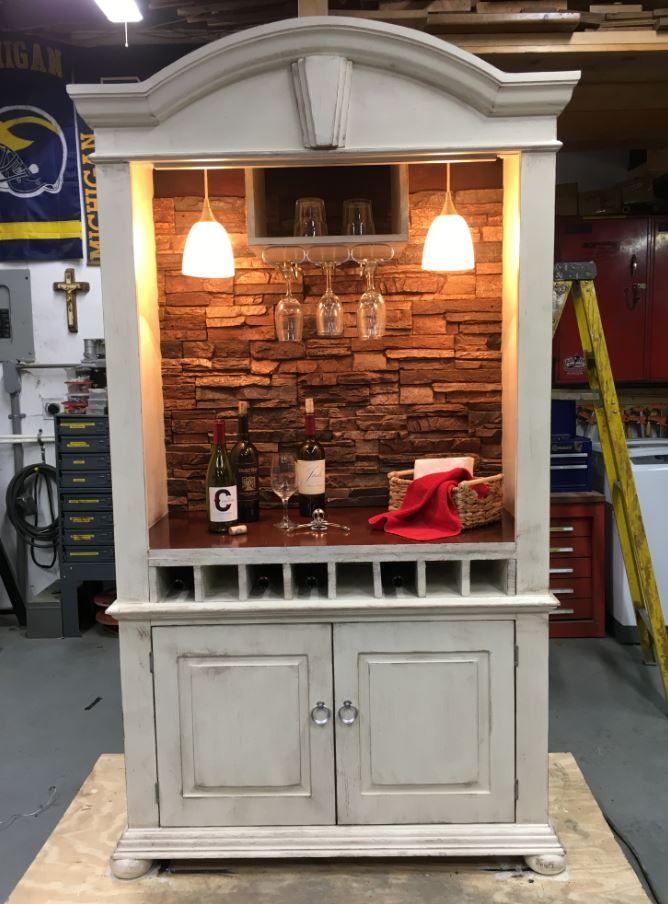The image depicts a repurposed white cabinetry, likely an old armoire or dresser, transformed into a sophisticated wine bar. Positioned centrally, the cabinetry features a stone wall backdrop that provides a rustic charm. Three wine bottles are displayed prominently on the counter, with wine glasses hanging from a rack beneath two installed lights, highlighting the setup. Additional features include a basket and a bottle opener. The surrounding environment, filled with tools and drawers, suggests that this bar is situated in a garage or workshop. A banner in the background proudly displays "Michigan," contributing to the personalized and cozy atmosphere. The color palette of the image includes red, blue, yellow, slate gray, and off-white, adding to its visual appeal.